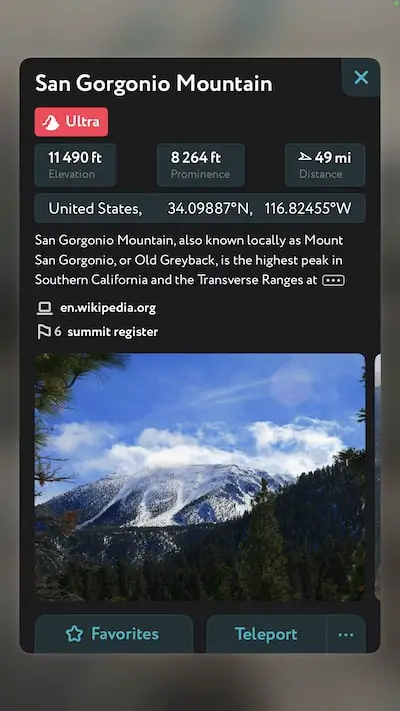The image displays a smartphone screen showcasing a picturesque mountain scene. The mountain, topped with snow and framed by drifting clouds, is identified at the top of the screen as San Gregonio Mountain. Just beneath this heading, within a bold red box, is the word "Ultra," followed by various details: an elevation of 11,490 feet, a prominence of 8,264 feet, a distance of 49 miles, and its coordinates of 34.09887° N, 116.82455° W in the United States. This information describes San Gregonio Mountain, also known locally as Mount San Gregonio or Old Grayback, which is the highest peak in Southern California and part of the Transverse Ranges.

Beneath these details, there is a Wikipedia icon accompanied by the URL "en.wikipedia.org." Adjacent to this is an icon of a flag with the text "Sixth Summit Register" next to it. Below this section, the central image of the mountain clearly highlights its snow-covered peak and surrounding scenery.

At the bottom of the screen, directly below the mountain image, there are two tabs. The first tab features a star icon with the label "Favorites" beside it. To its right, the second tab displays the text "Teleport..." Beyond these, there is no additional text or images present on the screen.